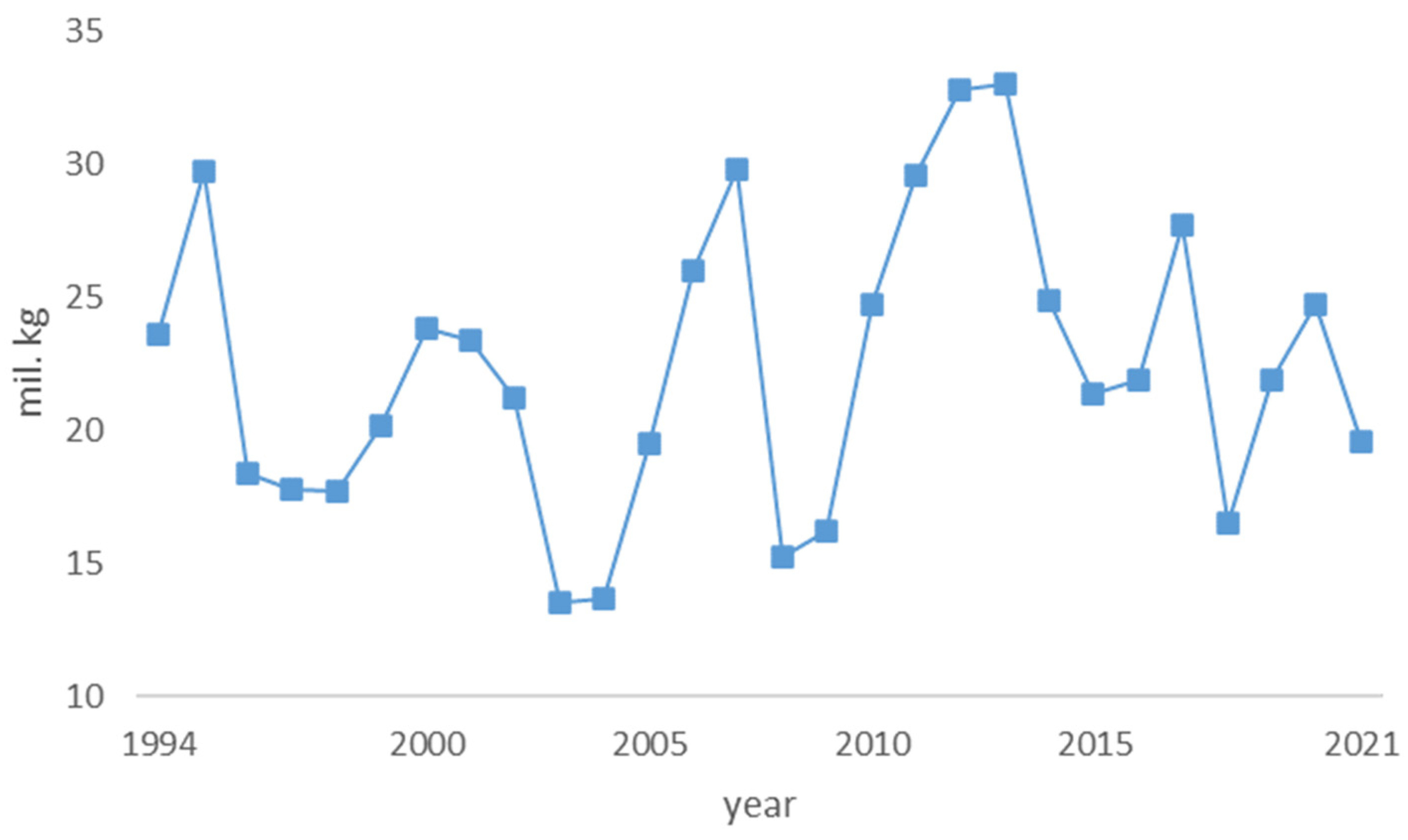The image displays a graph on a simple white background, with axes labeled in gray. The horizontal axis represents the years spanning from 1994 to 2021, with specific markers at '94, 2000, 2005, 2010, 2015, and 2021. The vertical axis, labeled "MIL.kg," ranges from 10 to 35. A light blue line with blue squares at data points charts the values year by year. The graph reveals significant fluctuations, peaking between approximately 2005 and 2012. Despite the representation, the graph does not specify what the measured values are, only showing that by 2021, the value is lower than it was in 1994.